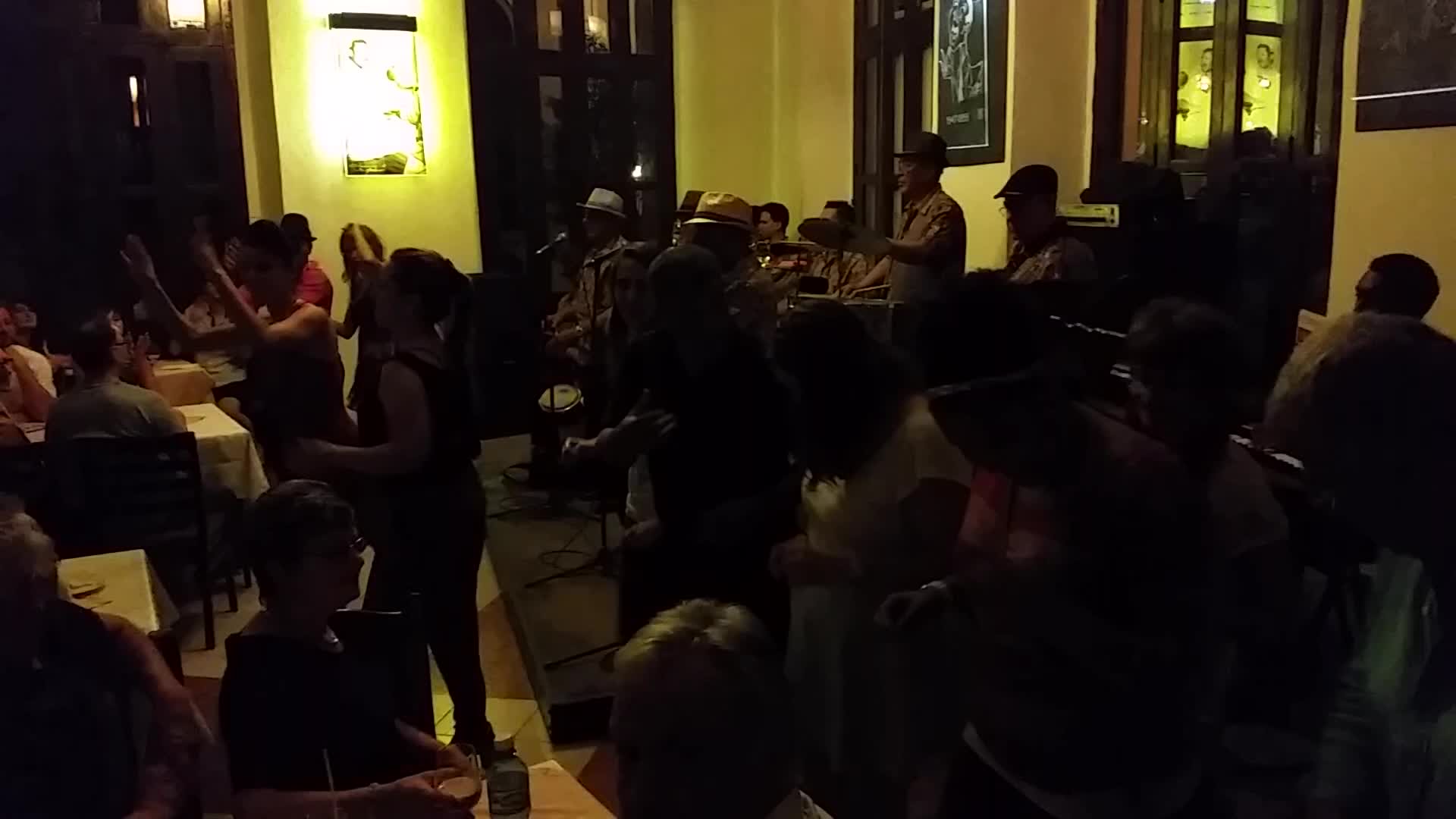The image depicts a dimly-lit restaurant or event venue at nighttime. The background features yellow-greenish walls with windows around the room. On the right-hand side, a band composed of mostly senior members is performing with various instruments, including drums, bongos, cymbals, and a guitar. In the foreground, three women stand with their hands raised, possibly dancing. To the left, patrons sit at tables, some clapping and dancing, while others enjoy the performance from their seats. Despite its darkness, the image captures a lively and engaging atmosphere with people immersed in the live music.